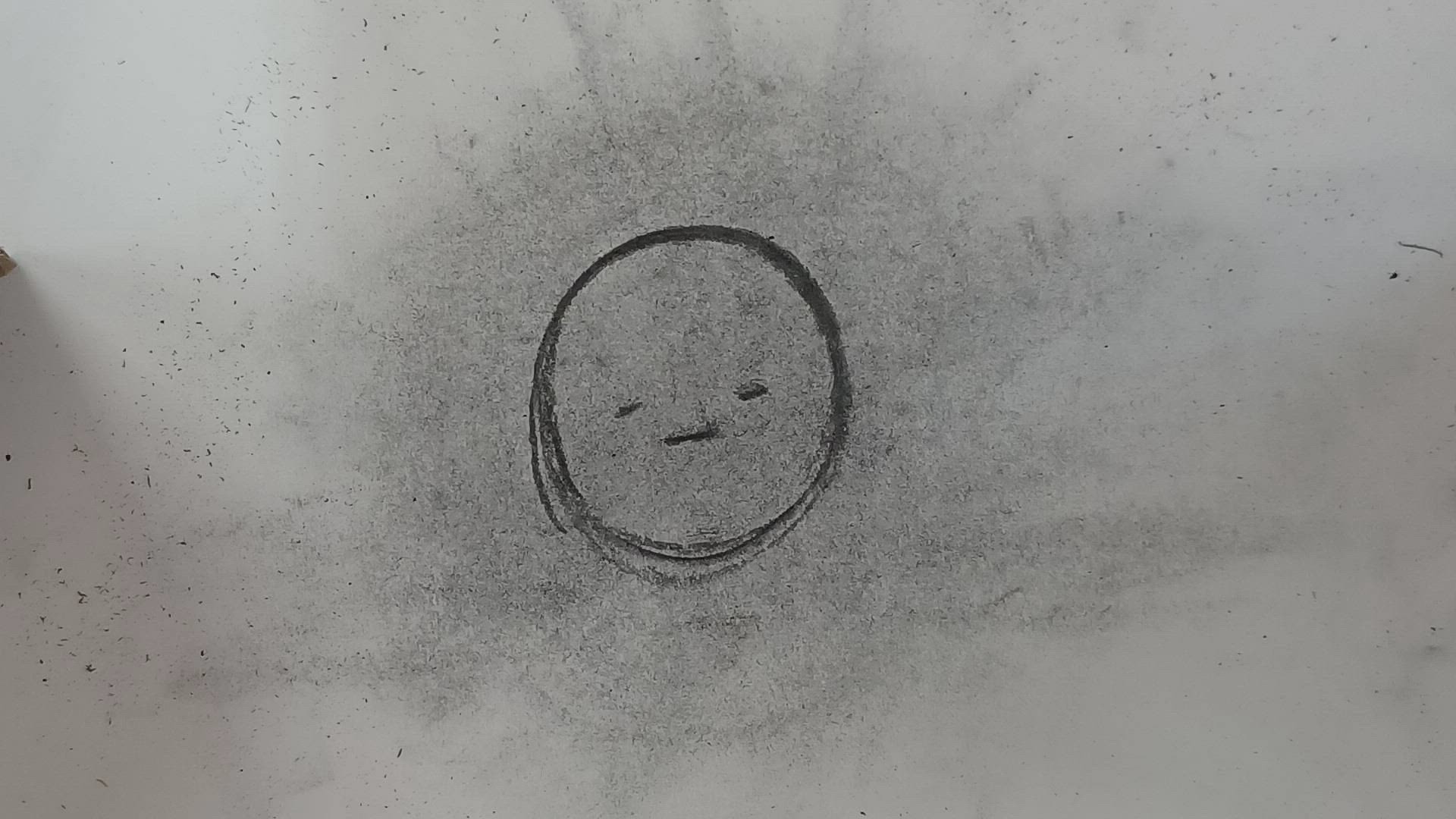The image is a pencil or charcoal drawing on a white piece of paper, capturing the simplistic likeness of a face. At the center of the page, there is a sketched circle approximately three to four inches in diameter. The circle is shaded in gray with varying thickness; the top of the circle has a thicker, darker outline which gradually becomes thinner towards the bottom. The head's rough texture suggests multiple attempts to draw the circle, overlapping to give a darker, smudged appearance typically associated with charcoal drawing.

The facial features are minimalistic: two short horizontal slits for eyes, each about a fourth of an inch long, and a horizontal line for the mouth measuring roughly an inch in width, giving the face a neutral expression. Charcoal smudges subtly shade the background of the face, contributing to a light gray aura surrounding the circle. Additional gray shading radiates from the top and sides of the head in ray-like extensions. Black dots sporadically mark the outer white space, along with a small line on the right side of the page, enhancing the drawing's textured, sketchy feel.